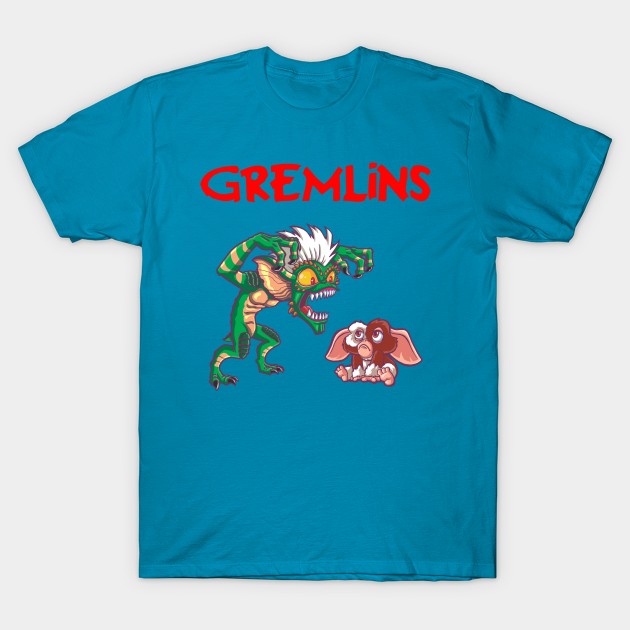This image showcases a teal blue t-shirt laid flat against a plain white background, likely intended for a product advertisement. The t-shirt features vibrant red lettering across the chest that reads "GREMLINS." Below the text, on the left side, is a detailed depiction of a green monster with a reptilian appearance. This creature has vibrant yellow eyes with red pupils, a tuft of white hair on its head, and large, sharp white teeth. It also has a gold-colored abdomen and wings, and it is standing upright on black webbed feet with claws, its arms raised menacingly in the air. To the right, a smaller gremlin-like creature sits on the ground with its legs extended and palms flat on the floor. This smaller figure is primarily brown with white patches and features large, pinkish ears and human-like feet. The detailed imagery and bold design elements make the t-shirt visually striking.